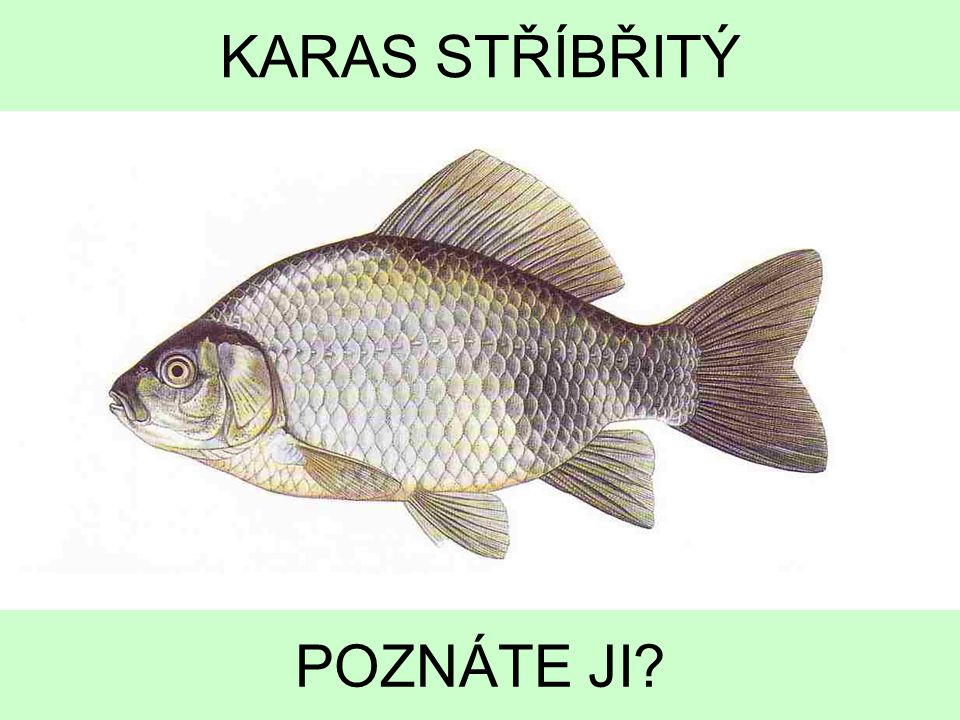The image displays a fish, which appears to be one you might catch in a lake or stream. The fish has a distinctive yellowish-silver coloration with brown and white accents. Its features, including its eye, fins, tail, scales, and mouth, are clearly visible. The fish is centrally positioned on a white background, with its body oriented horizontally from its mouth on the left to its tail on the right.

Above the fish, there's a green-bordered text box with the words "Karas Strabriti" written in an unfamiliar language. At the bottom of the image, there's a light green banner with the text "Pazneteji?" in black letters. The overall composition suggests this could be an educational page about fish, possibly from a book or a school resource.